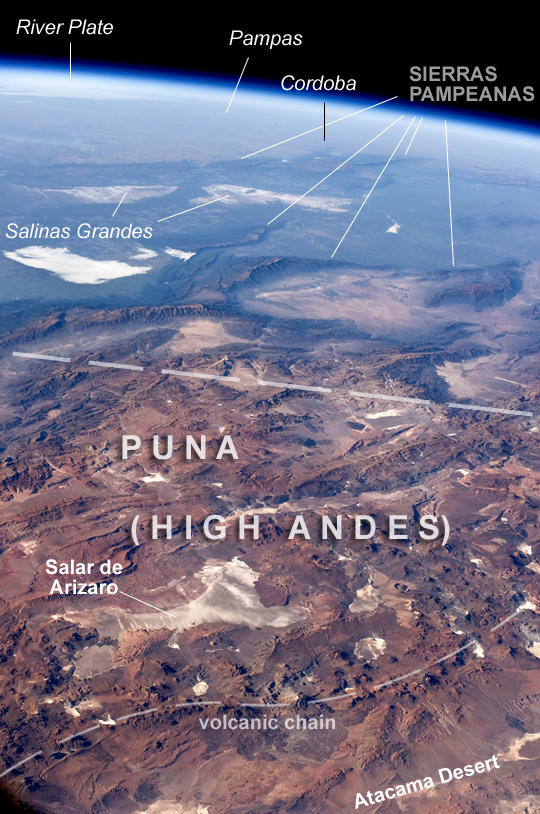The image is an aerial shot, likely from a plane, capturing the rugged landscape of the Puna region in the High Andes. The upper portion of the image is predominantly black, transitioning into grayed-out areas that highlight River Plate, Palmas, Cordoba, Sierra Pampanillas, and Salinas Grandes. Below these labels, the terrain features more brown hues, delineated by a white line, with the central label reading "Puna, High Andes" and "Salar de Arzerio". Another white line demarcates the area described as the "Volcanic Chain". In the lower right corner, text indicates the "Atacama Desert". Overall, the scene is a mix of brown, white, blue, light blue, and black tones, capturing the vast, mountainous expanse.